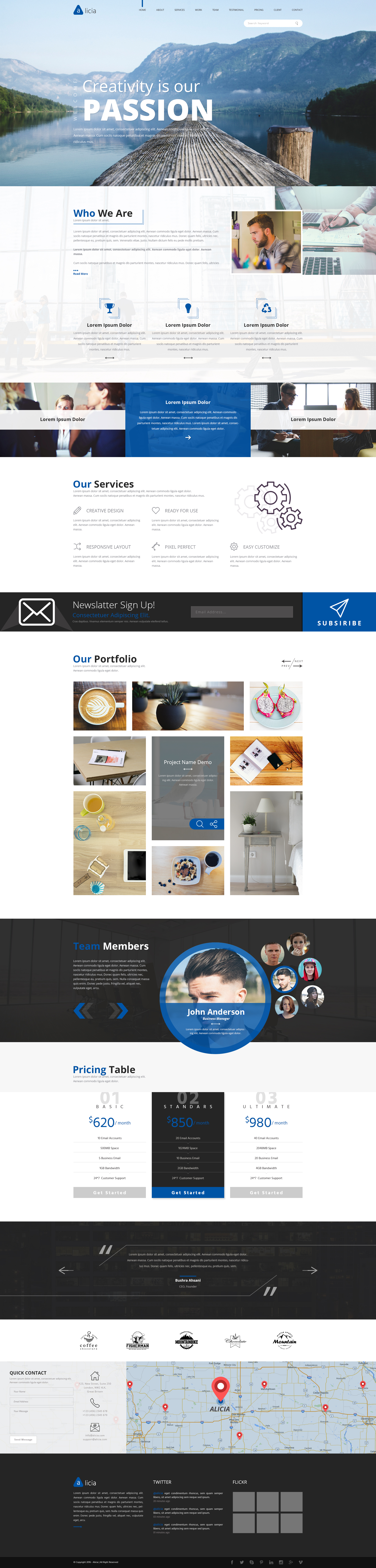This screenshot showcases an entire webpage, featuring a slightly blurred and stretched visual presentation. Dominating the top section, the page prominently displays the text, "Creativity is our passion," against a picturesque backdrop of mountains, water, and a bridge. 

Below this headline, the section titled "Who Are We?" appears, accompanied by a brief descriptive paragraph and two side-by-side media images. Further down, three small icons are visible, with one clearly depicting a trophy symbol, the others are indiscernible.

Centrally located, a prominent blue box with centered text starts with "Followed by our service," alongside an icon depicting cogs and additional information. 

Adjacent to this, the next section showcases an envelope and arrow icon, leading into the "Our Portfolio" area, which contains a variety of media images. Following this, the “Team Members” section highlights individuals with their photos encased in circles.

Near the bottom of the page, a section appears to display a map, likely indicating a GPS location, along with additional information that remains partially obscured at the very end of the screenshot.